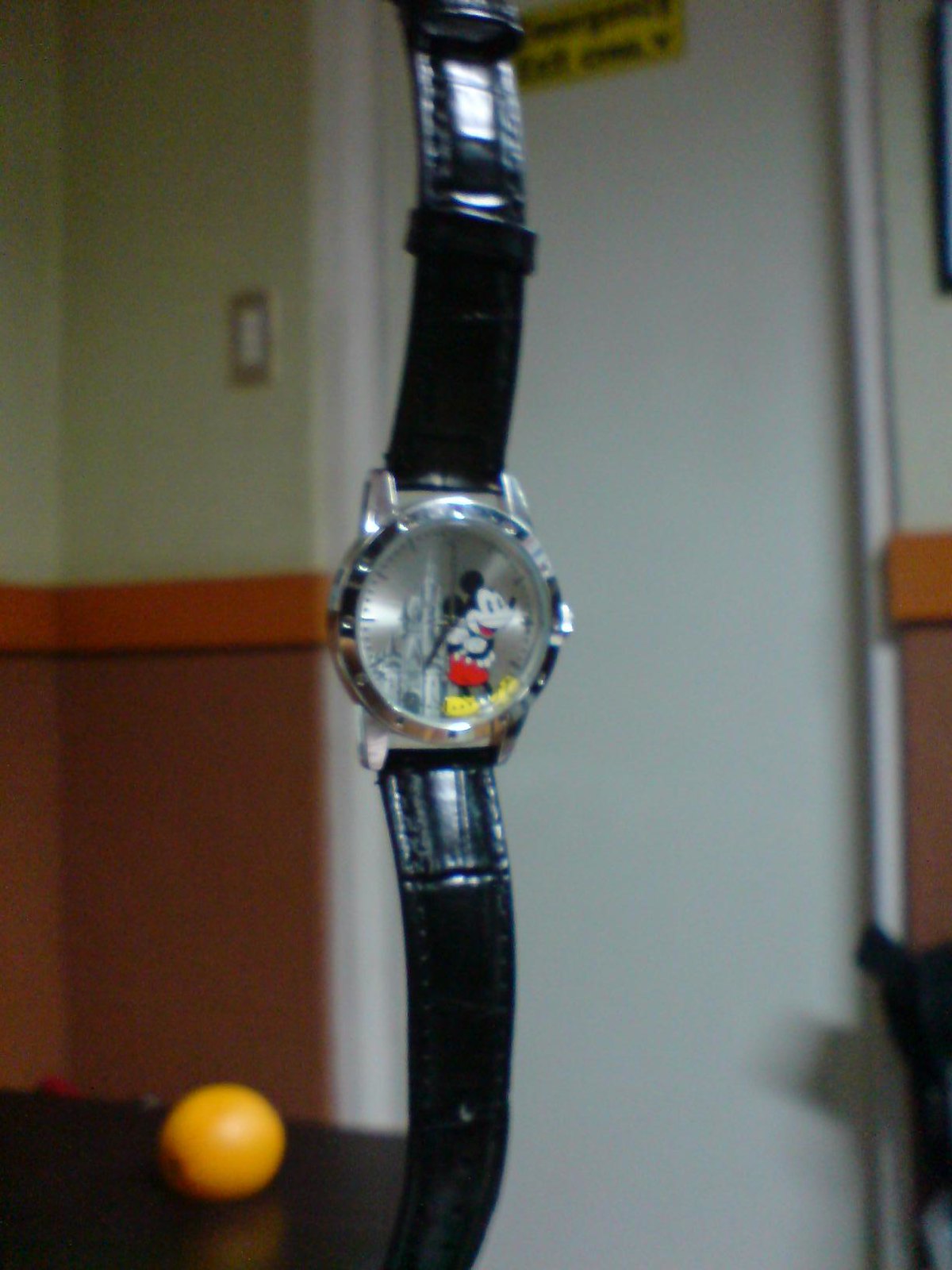This indoor photograph showcases a wristwatch being held up vertically in front of the camera, set against a distinctively detailed background. The bottom half of the room features rich wood paneling, while the upper half is painted a clean, crisp white. A white door can be seen in the background, alongside a dark wooden table that holds a bright orange, adding a pop of color to the setting. The watch's band is black, and it could be made of either real or faux leather, providing an elegant contrast to the rest of the watch. Its frame is crafted from silver, complementing the silver watch face which is adorned with a charming picture of the iconic Disney World castle. Adding a nostalgic touch, the face also features an old-fashioned Mickey Mouse character. The minute and hour hands are designed as sleek, needle-like rectangles, pointing to small dashes instead of traditional numbered markers, making this timepiece both functional and a delightful collector's item.